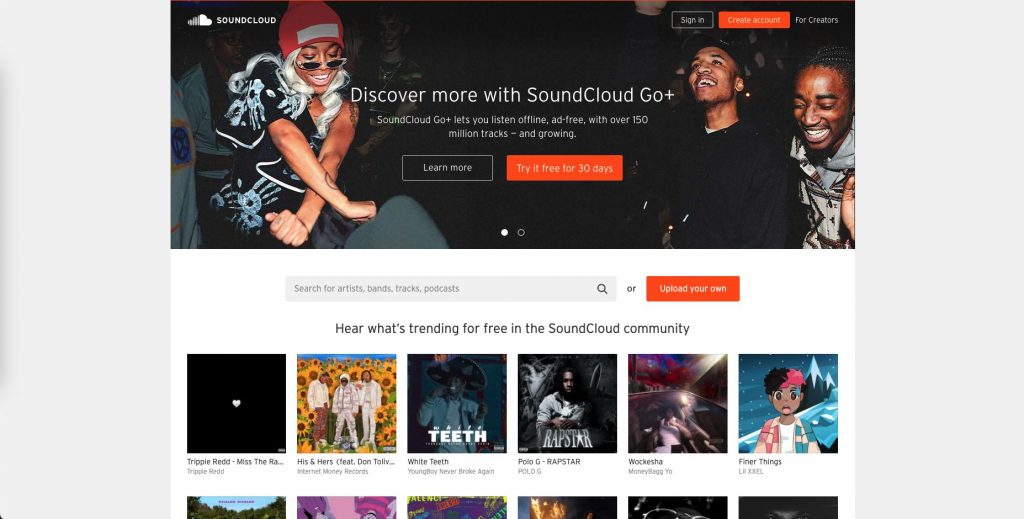Captured on a website, presumably SoundCloud, the top banner features an engaging scene. On the left, a woman dressed in a vibrant red beanie beams with joy, while on the right, two men share hearty laughter, creating an atmosphere of shared happiness. In the center of this banner, bold text invites users to "Discover more with SoundCloud Go Plus." Below this, two buttons are prominently displayed: one greyed-out button labeled "Learn More" and a striking orange button offering a "Try for free for 30 days" trial.

As we move further down the page, the interface showcases an array of music selections. Although the text is somewhat small, making it difficult to distinguish specific names, the layout is clear. The first box on the left is entirely black, save for a small white heart icon situated centrally. Below this, a series of six song listings and their accompanying images are neatly aligned. Another row of six songs follows beneath, although the image does not provide enough detail to identify them. This well-organized display hints at the rich musical experience awaiting exploration on SoundCloud.